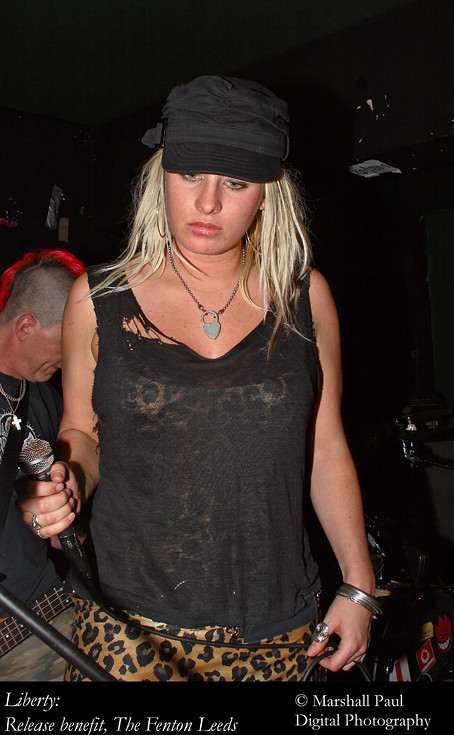In a dimly lit concert venue, a blonde woman stands on stage, facing forward with her head slightly bowed, giving her a contemplative look. She wears a black cap that partly obscures her long blonde hair, which cascades down to her shoulders, covering her ears. Her outfit exudes a rock band aesthetic, consisting of a black, ripped sleeveless tank top revealing glimpses of a leopard-patterned ensemble underneath. Leopard print pants complete her bold look.

She wears a necklace with a distinctive heart-shaped pendant. Adorning her hands are various silver rings, and on one wrist, she sports bangles. Her left hand hangs by her hip while her right hand holds a microphone at stomach level, suggesting she's either about to sing or has just finished a performance.

Next to her, a man with a striking red-tipped mohawk and short black hair sits, holding a guitar. He wears a black shirt and a necklace with a cross pendant. The backdrop behind them is almost entirely black, dotted here and there with small spots of white, accentuating the concert's shadowy atmosphere. At the bottom of the photo, a black bar displays the text: "Liberty Release Benefit, The Fenton Leeds, Copyright Marshall Paul, Digital Photography."